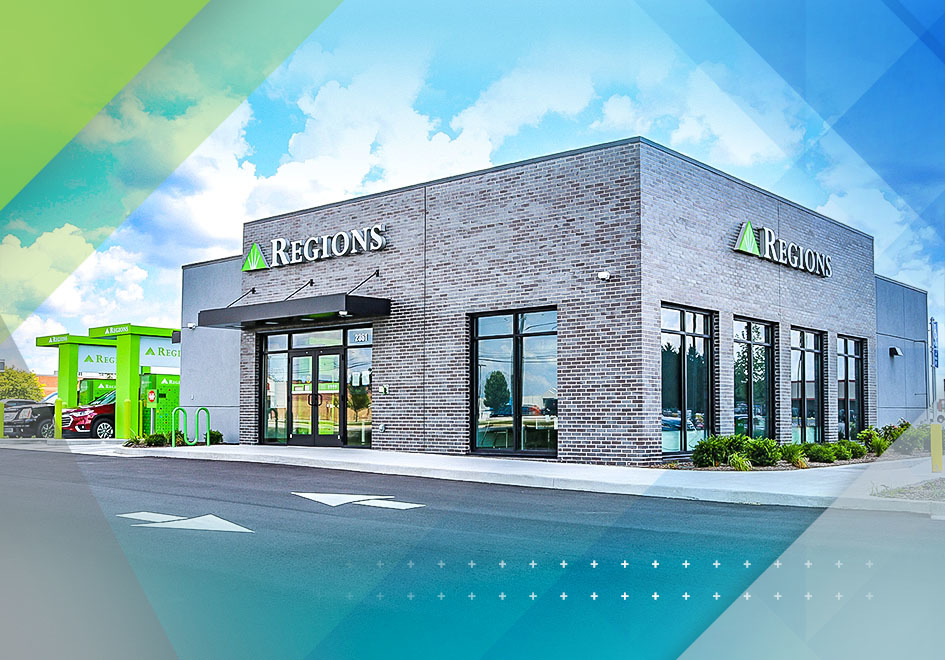This is a color photograph of a Regions Bank branch. The building is made of square brick and features windows halfway up its sides. Prominently displayed above the windows are signs that read "Regions" in white, accompanied by a distinctive lime-green triangle logo. The image captures a clear view of the bank’s front door and part of the side, highlighting the drive-in area to the right. This area, including drive-up windows and ATMs, is marked by the same green color as the bank’s logo.

The bottom half of the photograph shows several features: a red car and a black car are currently situated at the outdoor teller windows. There are lime-green marked parking spots at the back of the building, and a green bike rack is positioned in front. The landscaping around the bank includes small green bushes. The sky is a clear blue with scattered white clouds, and the image has a stylistic touch with diagonal bands of color at each corner: green at the top left, blue at the top right, dark gray at the bottom left, and light gray at the bottom right.